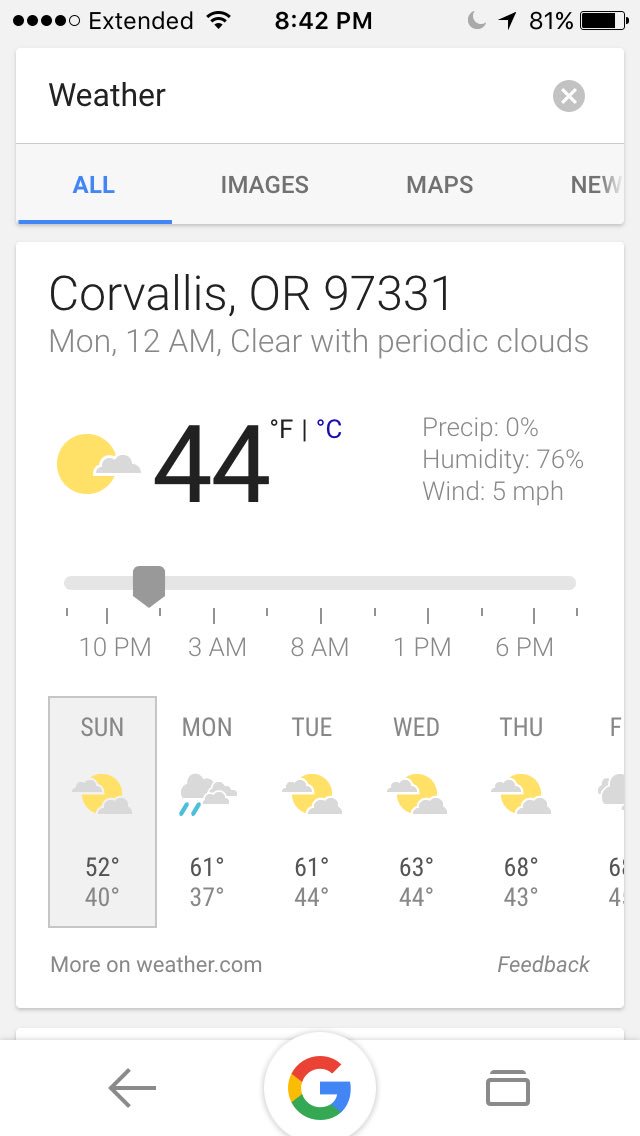The image showcases a smartphone interface in portrait mode, displaying a weather application. At the top left corner, there is the text "Extended" next to a Wi-Fi symbol. The current time, 8:42 PM, is displayed prominently in black at the top center, while the top right corner features a moon icon, a black arrow, and a battery indicator showing 81%.

Below this header, the app displays several tabs: "All," "Images," "Maps," and "News," with "All" underlined in blue. The central part of the screen is dedicated to weather information for Corvallis, Oregon, 97331. Highlighted in gray, it indicates the conditions for Monday at 12 AM: "Clear with periodic clouds." The main temperature reads 44°F in large black text, accompanied by a clickable Celsius icon.

An icon representing the current weather—a moon with a cloud—appears adjacent to the temperature. To the right, additional details include "Precipitation 0%," "Humidity 76%," and "Wind 5 mph." A bar at the bottom illustrates hourly weather forecasts, while a weekly forecast below spans Sunday through Friday, showing daily weather icons and temperatures.